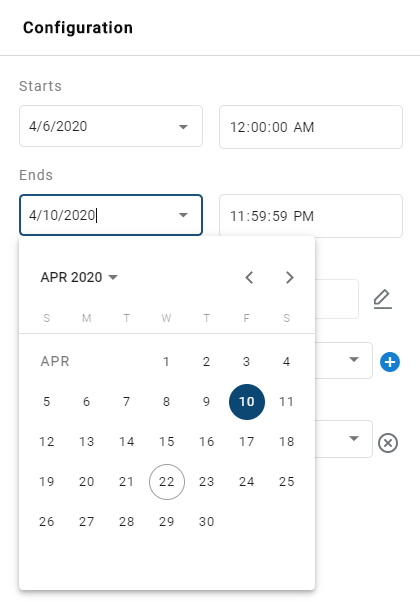This is a cropped screenshot of an alert configuration screen featuring a clean white background. In the top left corner, the word "Configuration" is prominently displayed in bold black font, separated from the rest of the interface by a thin gray line. Below this line, on the left-hand side, the label "Starts" appears in bold gray font. Underneath "Starts," there's a drop-down box set to April 6, 2020, with an adjacent time box displaying 12:00 AM. 

Further down, the label "Ends" is also shown in bold gray letters. Directly below this, another drop-down box indicates an end date of April 10, 2020. An open calendar box beneath this shows April 2020 at the top, with the 10th highlighted by a blue bubble, signifying its selection. To the right of the end date, the time is set precisely to 11:59:59.

Additionally, the right edge of the screenshot reveals parts of three other text boxes or drop-down boxes positioned vertically. Each of these elements is accompanied by a corresponding icon on the left side, hinting at further configuration options just outside the visible area.